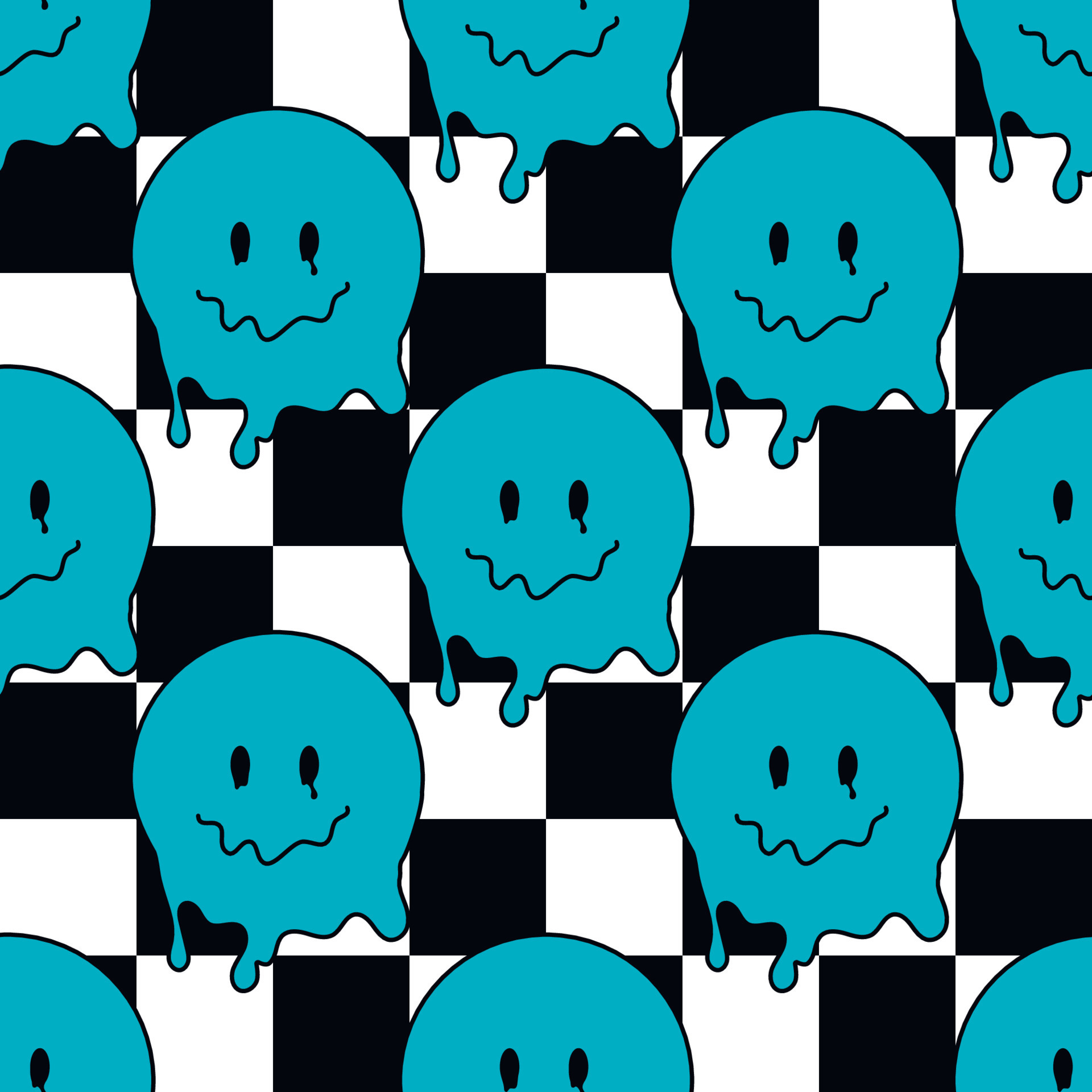The image features a detailed black and white checkerboard pattern, consisting of eight squares across and eight squares down, beginning with a white square in the top-left corner and alternating consistently. Superimposed on this checkerboard are twelve moodily designed smiley faces in a dull aquamarine or teal color. These smiley faces, sized to cover an area of four squares, have perfectly circular tops but appear to be melting or oozing downwards, with dripping lower edges and droopy black oval eyes. Their crooked, wiggly smiles add to their forlorn appearance, as if they are slowly melting away. Arranged symmetrically across the checkerboard, the smiley faces form a pattern with rows of three, two, three, two, and three from top to bottom, creating a visually engaging contrast with the stark checkerboard background.